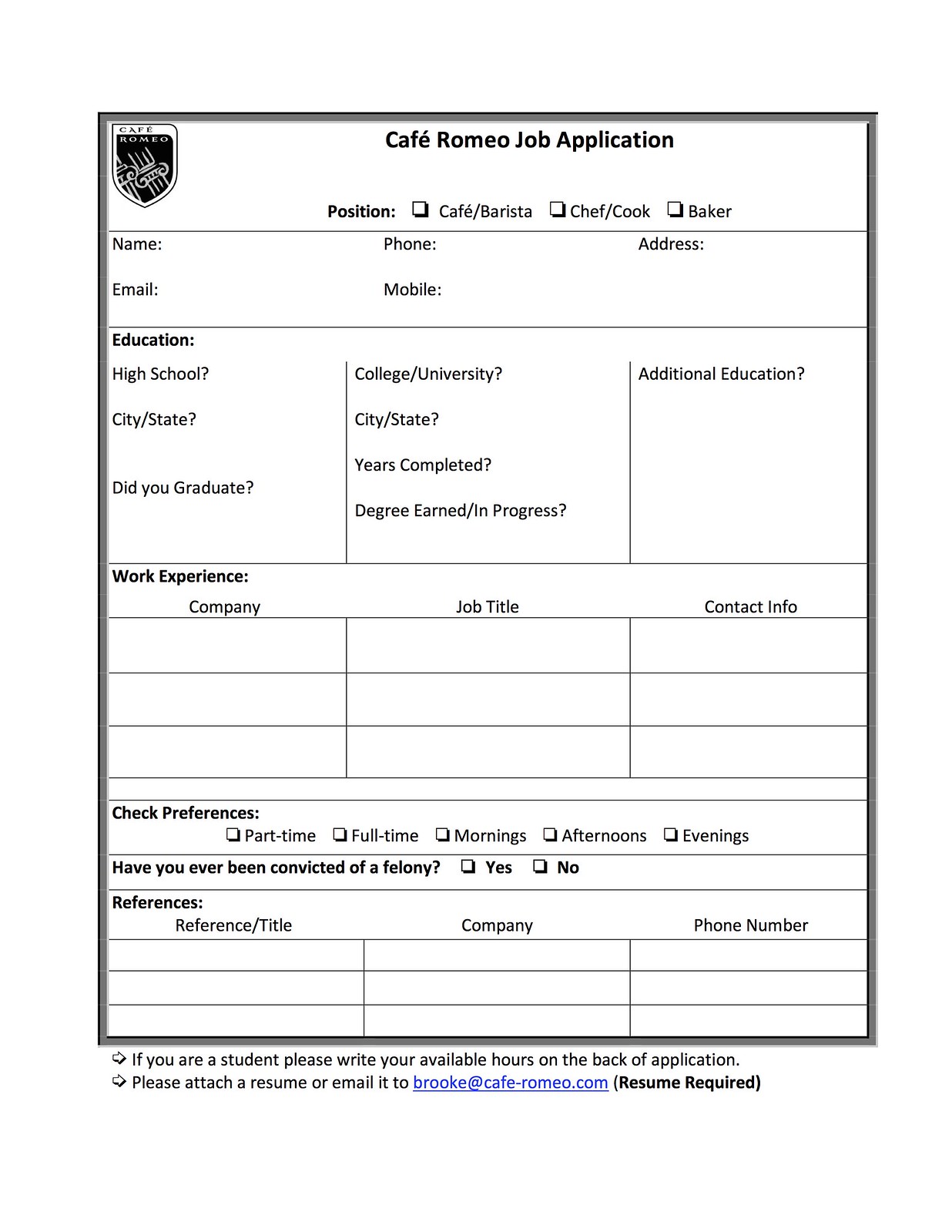The image is a detailed screenshot, or possibly a photocopy, of a PDF file displaying a job application form for Cafe Romeo. In the top left corner, there is a symbol, followed by a large title that reads "Cafe Romeo Job Application." Below the title, the form is divided into various sections by dark lines. The first section includes checkboxes for the desired position—Cafe, Barista, Chef, Cook, or Baker.

Following that, there are fields for personal information, including spaces for the applicant's name, phone number, address, email, and mobile phone. The subsequent section is dedicated to educational background, with fields for high school and college/university information such as city, state, graduation status, years completed, and degree earned or in progress. An additional column is provided for any other educational qualifications.

Next, the form has a section to list work experience, asking for the company name, job title, and contact information. There are checkboxes for the applicant to indicate their work preferences, such as part-time or full-time and specific shift availability—mornings, afternoons, or evenings. Following this, there is a question about felony convictions with yes or no checkboxes.

The references section is included next, requiring details like reference name, company, and phone number. At the bottom, there is a note instructing students to write their available hours on the back of the application and to attach a resume or email it to brook at cafe romeo dot com, with the parenthetical note stating "resume required."

The overall color scheme of the form is white, gray, black, and blue, occupying the entirety of the image without any additional objects, making it clear and straightforward for someone applying for a job at Cafe Romeo.